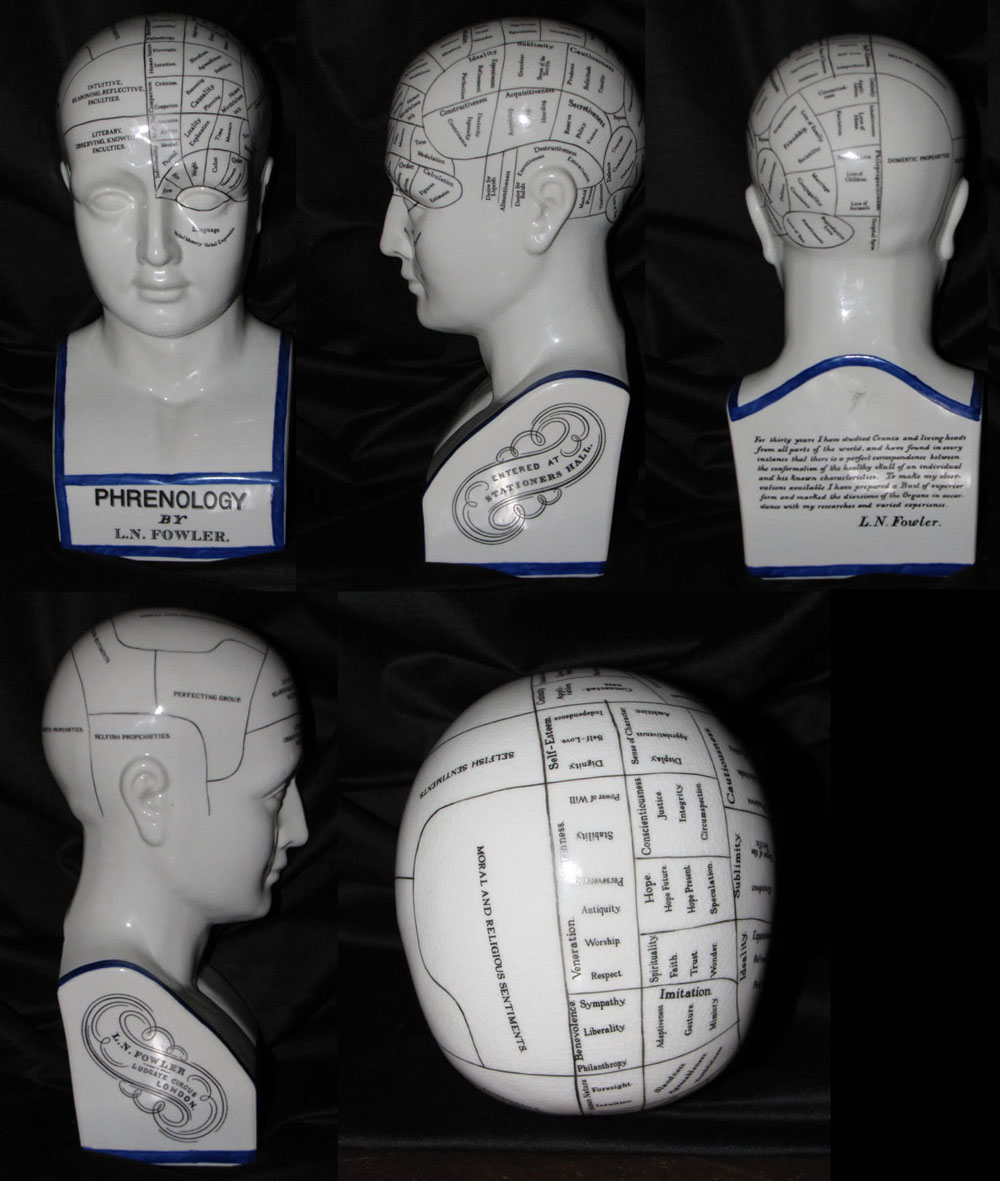The image displays a detailed instructional model of a phrenological dummy head, showcasing various segments of the skull and brain with black markings and labels. The white bust features noticeable black text and lines demarcating different regions of the head as per phrenology principles. Centrally labeled on the front of the chest is "Phrenology by L.N. Fowler" in distinct black text, and on the right side of the head, it reads "L.N. Fowler, Ludgate Circus, London." The back of the head is covered in text that is too blurred to read. The image is set against a black fabric background and includes five photographs of the same model from multiple angles. The top row consists of three views: the front-facing head, the left side profile, and the back of the head. The bottom row features two more: the right side profile and an enlarged top view of the head. Each perspective highlights the meticulously labeled sections believed to correspond with different personality traits. The rectangular image, approximately five inches tall and four inches wide, captures the bust from the upper chest upwards, emphasizing its educational purpose in phrenology.